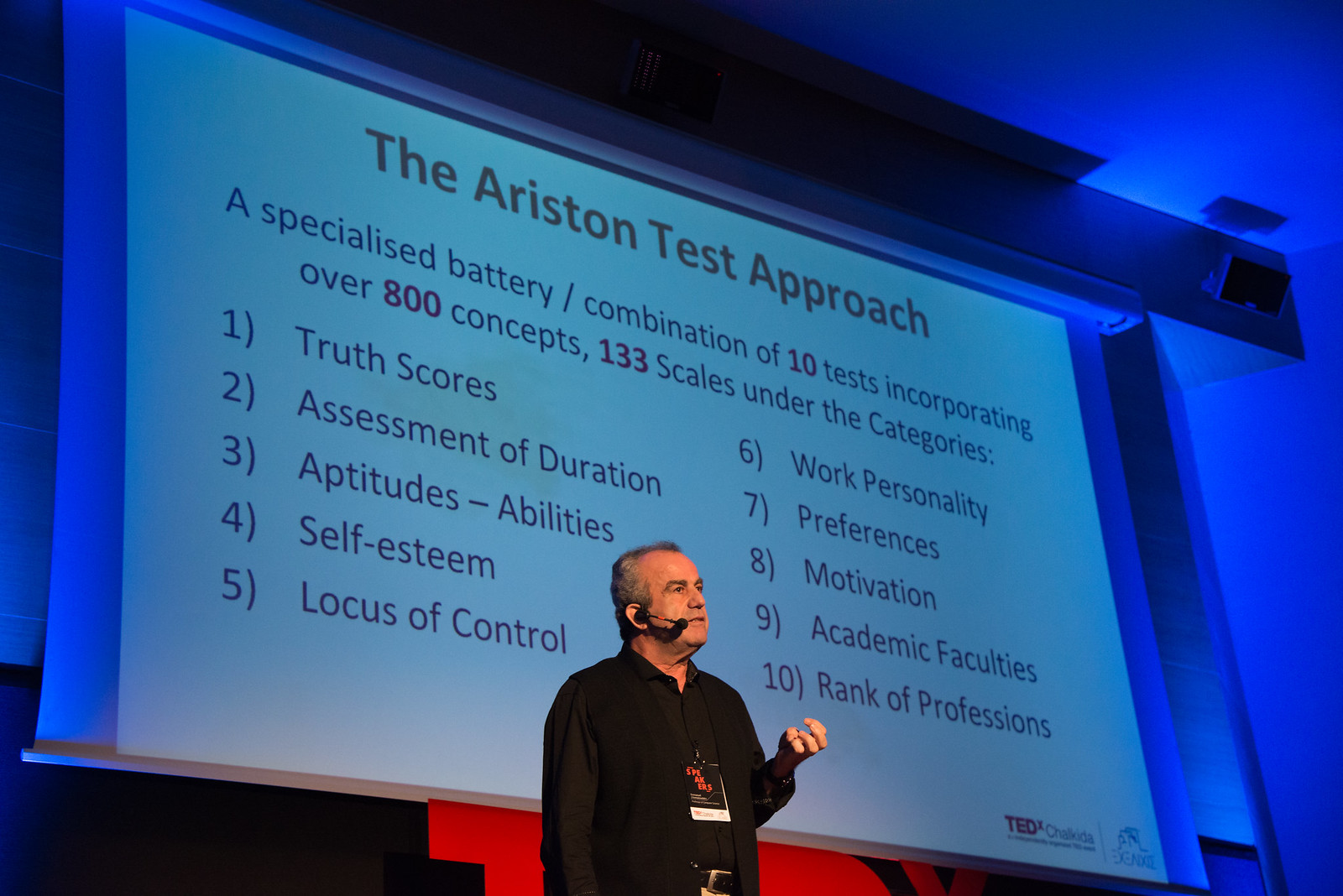In the image, a man is captured mid-presentation on a stage, giving what appears to be a TEDx talk, as indicated by the "TEDx" logo in the lower right corner of the projected slide behind him. He is attired in a long-sleeved, all-black button-down shirt and wears a badge, suggesting he is part of an organized event. His voice is amplified through a headset microphone, which is small and discreet. The stage is dramatically lit with blue and red lights, creating a vivid background. The speaker is making an expressive gesture with his left hand, emphasizing a point to the audience, which is out of the frame.

Behind him, a large screen dominates the center of the image, displaying a slide titled "The Ariston Test Approach." The content of the slide details a specialized battery of 10 tests that incorporate over 800 concepts and feature 133 scales. These tests are categorized into truth scores, assessment of duration, aptitudes, abilities, self-esteem, locus of control, work personality preferences, motivation, academic faculties, and rank of professions. The colors in the scene include black, red, orange, white, blue, and gray, contributing to the professional and engaging atmosphere of the presentation.